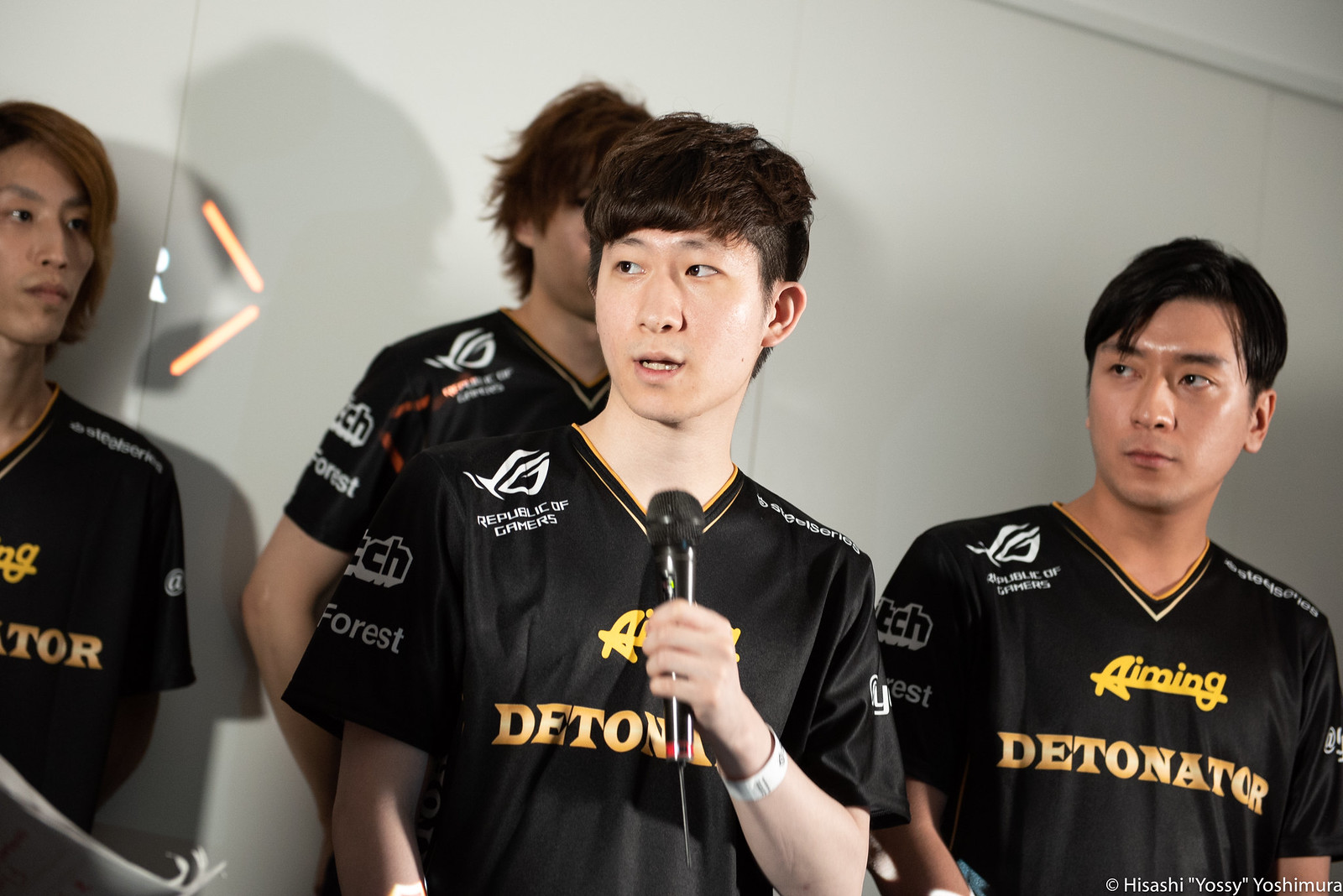The image depicts four young men, likely of Japanese or Asian descent, dressed in black sports uniforms with yellow and white designs. These uniforms bear the team name "Aiming Detonator" along with a symbol in the top left corner reading "Republic of Gamers." Three of the men have brown hair, including the one in the middle who is holding a microphone, suggesting he is speaking, perhaps giving an interview or speech. The man on the right has black hair while the one on the left has blonde hair. They stand against a plain white wall, which also features two small orange symbols. The man in the center additionally sports a white bracelet.